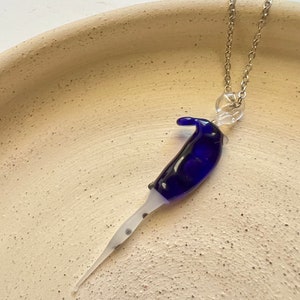The image showcases a seahorse-shaped pendant placed on a rough-textured, tan terracotta tray with a circular shape, resembling a shallow bowl. The pendant is crafted from glass and features a vibrant blue head transitioning into a semi-transparent white body dotted with small black spots, tapering to a sharp, wave-like point. This pendant is attached to a delicate gold chain, only partially visible in the upper right corner of the photo. The overall impression is of an intricately designed seahorse charm that combines elements of an icicle or stalactite in its form, highlighted by the contrasting colors and textured setting.